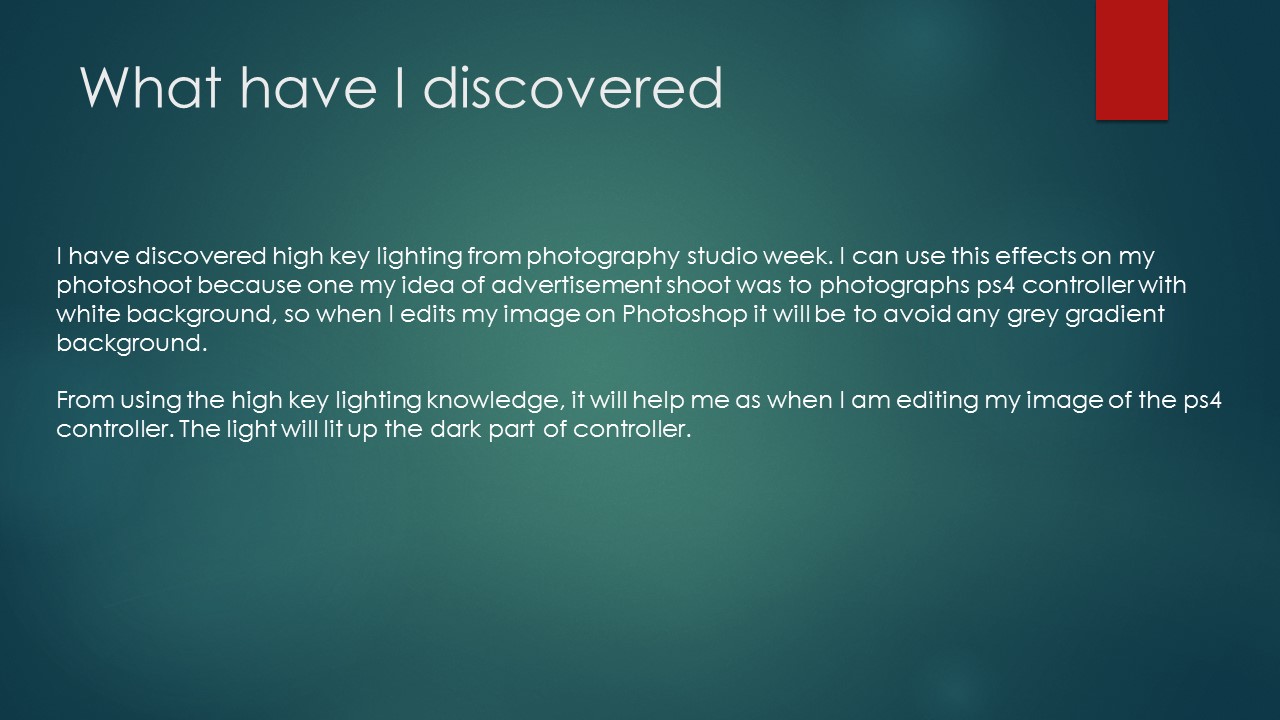The image portrays a small rectangular green card set against a teal background. The card is primarily green with some areas so dark they are almost black. The top of the card features a large title in white lettering: "What have I discovered?". Below the title, there are two paragraphs in smaller white text explaining a photography technique the author has learned. The text reads: "I have discovered high-key lighting from Photography Studio Week. I can use this effect in my photo shoot because one of my advertisement ideas was to photograph a PS4 controller against a white background. By using high-key lighting, I can avoid any gray gradient when editing the image in Photoshop, ensuring the light evenly illuminates the dark parts of the controller." In the upper right corner, a small red rectangle, resembling a ribbon or banner, hangs about an inch from the top. The card appears to be a student's work, possibly part of a thesis or a project submission, showcasing learning and application of photography techniques.